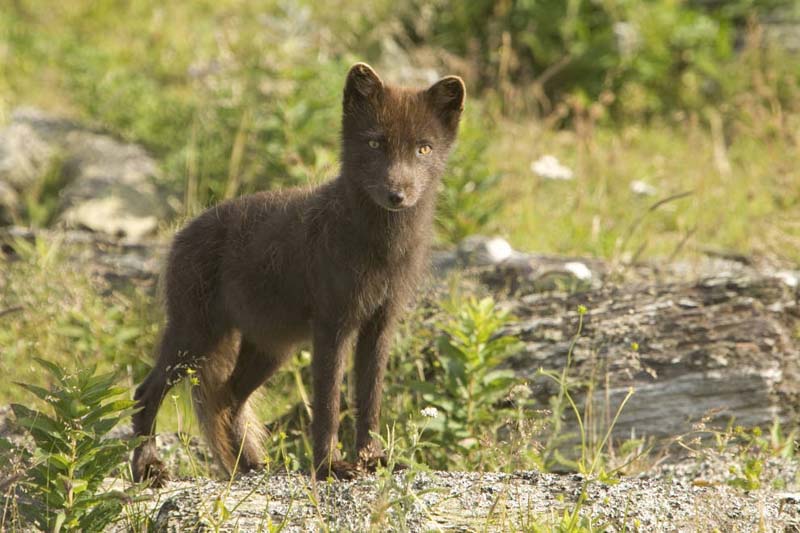The image captures a close-up of a young, wild canine, possibly a fox or a wolf, looking directly at the camera with striking yellow eyes. The animal is standing on a mix of grass and a gravelly, rock-strewn platform, with its dark grayish-brown fur contrasting against the vivid green surroundings. Sunlight streams onto the scene, highlighting the natural elements in the background, which include dense greenery, bushes, and patches of grass interspersed with scattered rocks. In the bottom left corner, plants add to the lushness of the setting, while a large fallen tree trunk is prominently positioned to the right. The overall impression is one of natural wilderness, with the young animal appearing curious and alert in its outdoor habitat.